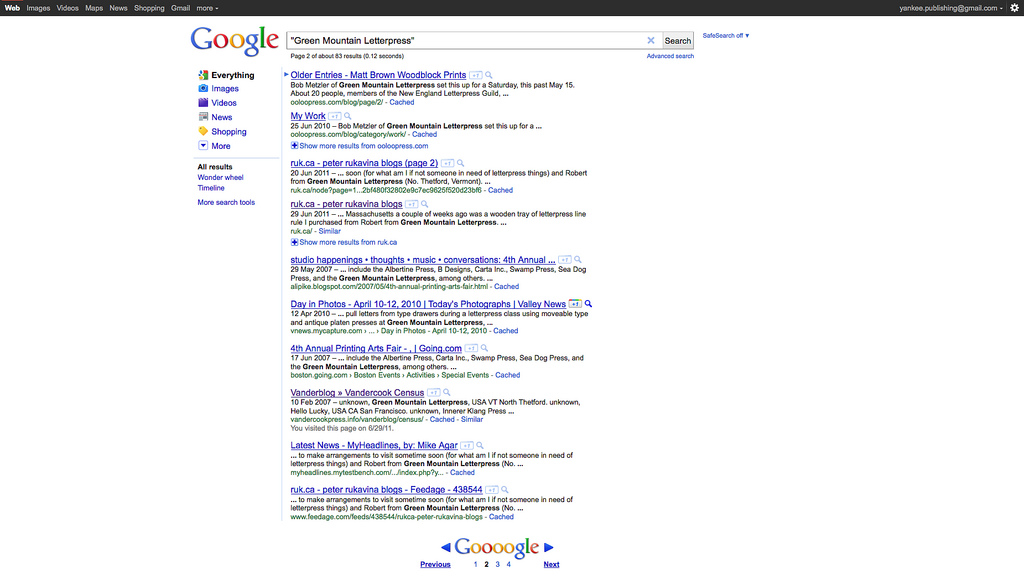This image is a landscape-oriented screenshot of a Google search results page. The screenshot appears to be taken on a desktop or laptop screen.

### Description:

In the **upper left** corner, a black horizontal bar features several Google service options: "Web," "Images," "Videos," "Maps," "News," "Shopping," "Gmail," and "More."

In the **upper right** corner, there is a partial view of an email address, ending with "@gmail.com," though some of the characters are unreadable.

At the **center top** of the page, there is a Google search bar containing the query: `"green mountain letterpress"`. Below the search bar, there is a horizontal sub-menu listing: "Everything," "Images," "Videos," "News," "Shopping," "More," with a down arrow indicating a dropdown menu for additional search tools.

The **left sidebar** presents various search refinement options: "All results," "Wonder wheel," "Timeline," and "More search tools."

In the **main body** of the page, the search results are displayed as follows:

1. **"Older entries"** - possibly indicating a link to previous posts or older search results.
2. **Matt Brown: Woodblock Prints** - likely a webpage or article related to woodblock prints by Matt Brown.
3. **My Work** - potentially a personal portfolio or projects page.
4. **ruk.ca: Peter Rukavina's Blog** - a link to Peter Rukavina's blog, specifically focusing on his writings and insights.
5. **ruk.ca: Peter Rukavina's Blog** - another link to Peter Rukavina's blog, perhaps a different post or section.
6. **Studio Happenings** - likely a blog or page detailing events and updates from a studio.
7. **Day in Photos: Fourth Annual Printing Arts Fair** - a photo gallery or blog post covering the Fourth Annual Printing Arts Fair.
8. **Vanderblog at Vanderbox Census** - a blog post or article from the Vanderblog, related to the Vanderbox Census.
9. **Latest News: My Headlines** - a collection of the latest news or personal highlights.
10. **ruk.ca: Peter Rukavina's Blog** - yet another link to Peter Rukavina's blog possibly leading to a specific entry or series of posts.

At the **bottom of the page**, page navigation is indicated with multiple page numbers. The number "2" is highlighted in black, denoting the current page, while the other numbers are displayed in blue, suggesting that they are clickable links to other pages.

Several links are shown in **purple**, indicating they have been previously visited:
- The **fourth link** ("ruk.ca: Peter Rukavina's Blog").
- The **third from the bottom** ("Vanderblog at Vanderbox Census").

This detailed caption provides a comprehensive description of the screenshot, structured to reflect both the layout and content of the search results page.